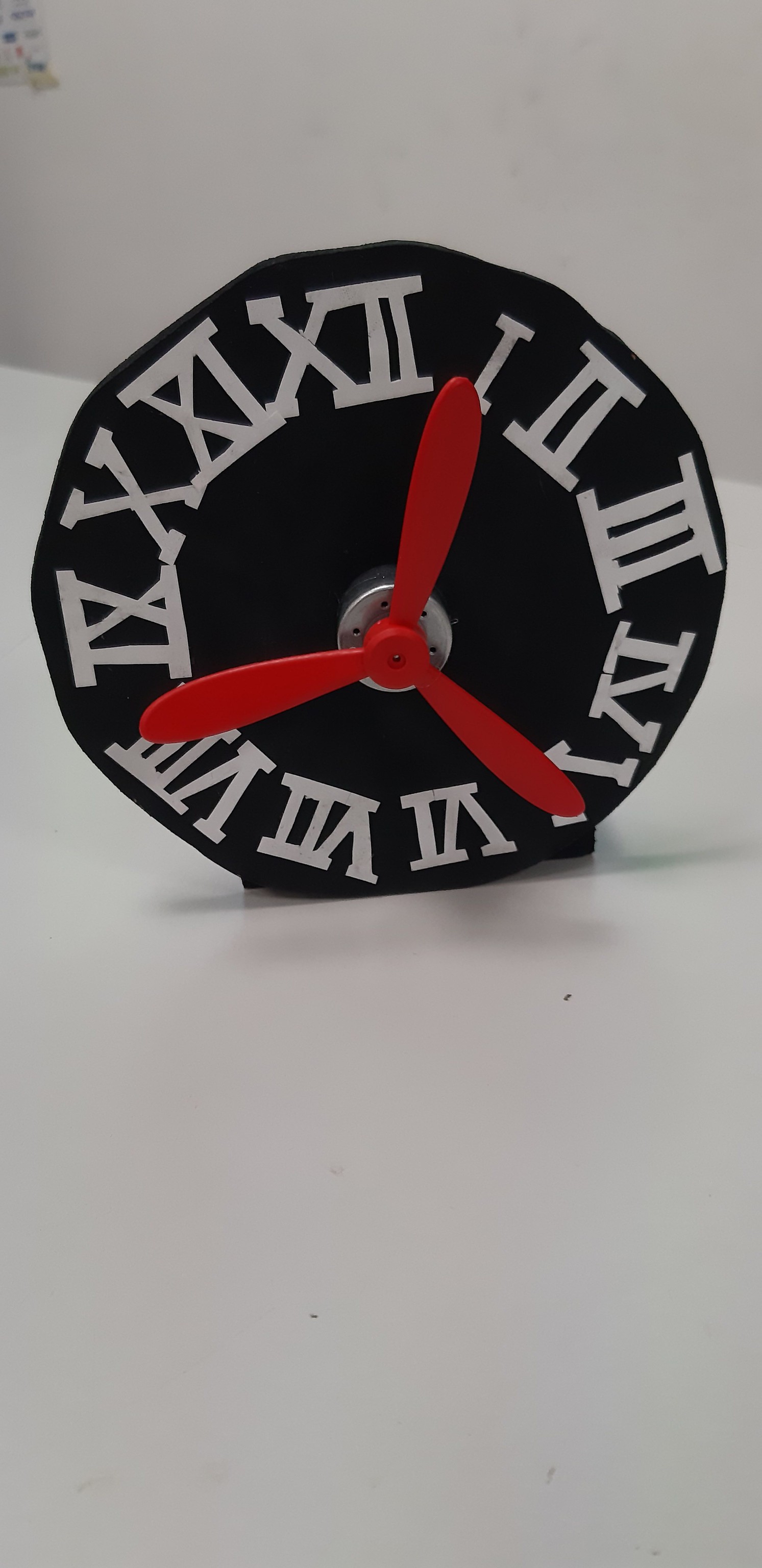This image captures a whimsical, irregularly-shaped clock set against a white background with a faint, slightly gray shading. The clock's face is predominantly black, marked with large white Roman numerals around its edge. The unique feature of this clock is its three hands, which are actually a red propeller mounted centrally on a silver washer, giving it an artistic and unconventional appearance. The clock appears to be resting on a round steel platform with a couple of hole perforations on the top surface, emphasizing its blend of functionality and creative design. The propeller serves as the minute hand, hour hand, and second hand in a triad formation, making this piece a striking blend of timekeeping and art.